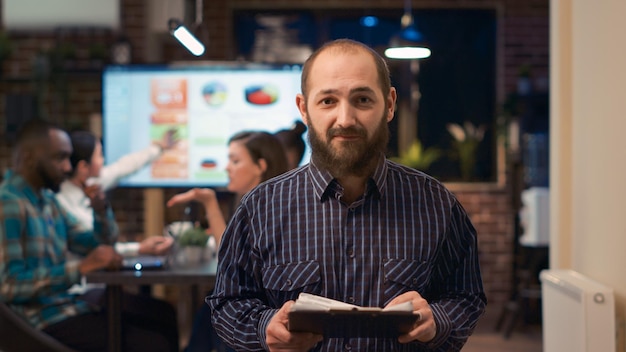In this indoor photograph, a man stands at the center holding a clipboard with several white papers in both hands. He is wearing a long-sleeved, collared, dark blue dress shirt adorned with light blue vertical and subtle horizontal stripes. The man has a full beard, a mustache, and is balding on the top of his head with remaining dark brown hair on the sides.

Behind him to the left, a group of four people are engaged in conversation around a table. One person from the group is pointing towards a large monitor displaying pie charts, though the details are blurry and indistinct due to the focus. To the right in the background, there are some shelves and what appears to be a paper shredder. The overall background is out of focus, adding a sense of depth to the image.